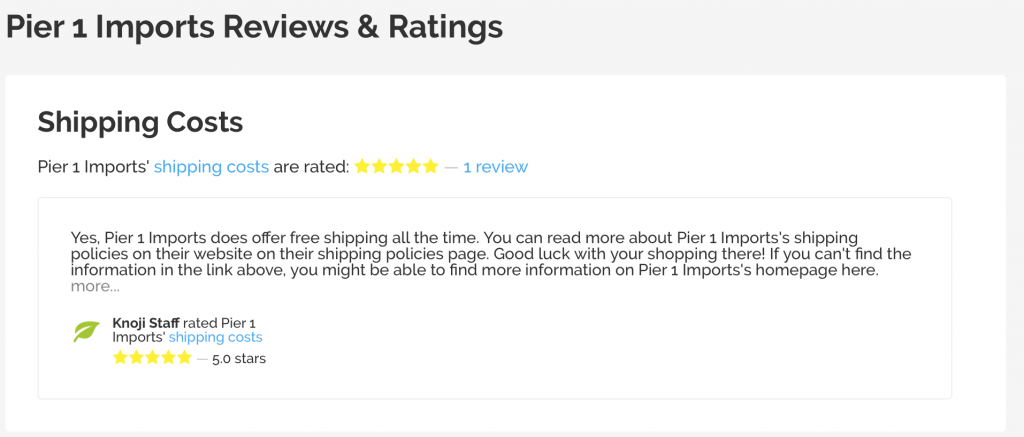**Caption:**

In this screenshot, the gray box at the top indicates the section title "Pier 1 Imports, Reviews, and Ratings." Below, the content is displayed on a white background. The main title, "Shipping Cost at Pier 1 Imports," is prominently featured in blue text. It is noted that the shipping cost has been rated 5 stars based on a single review.

The detailed review states that Pier 1 Imports consistently offers free shipping. For more comprehensive information on their shipping policies, readers are advised to visit the Pier 1 Imports website, specifically their Shipping Policies page. The review ends with encouragement to continue shopping and a suggestion to check the homepage for additional details if necessary.

The review is authored by a user with a green leaf icon next to their name, identified as "Kenoji Staff." This reviewer has given Pier 1 Imports' shipping cost a perfect score of five golden stars.